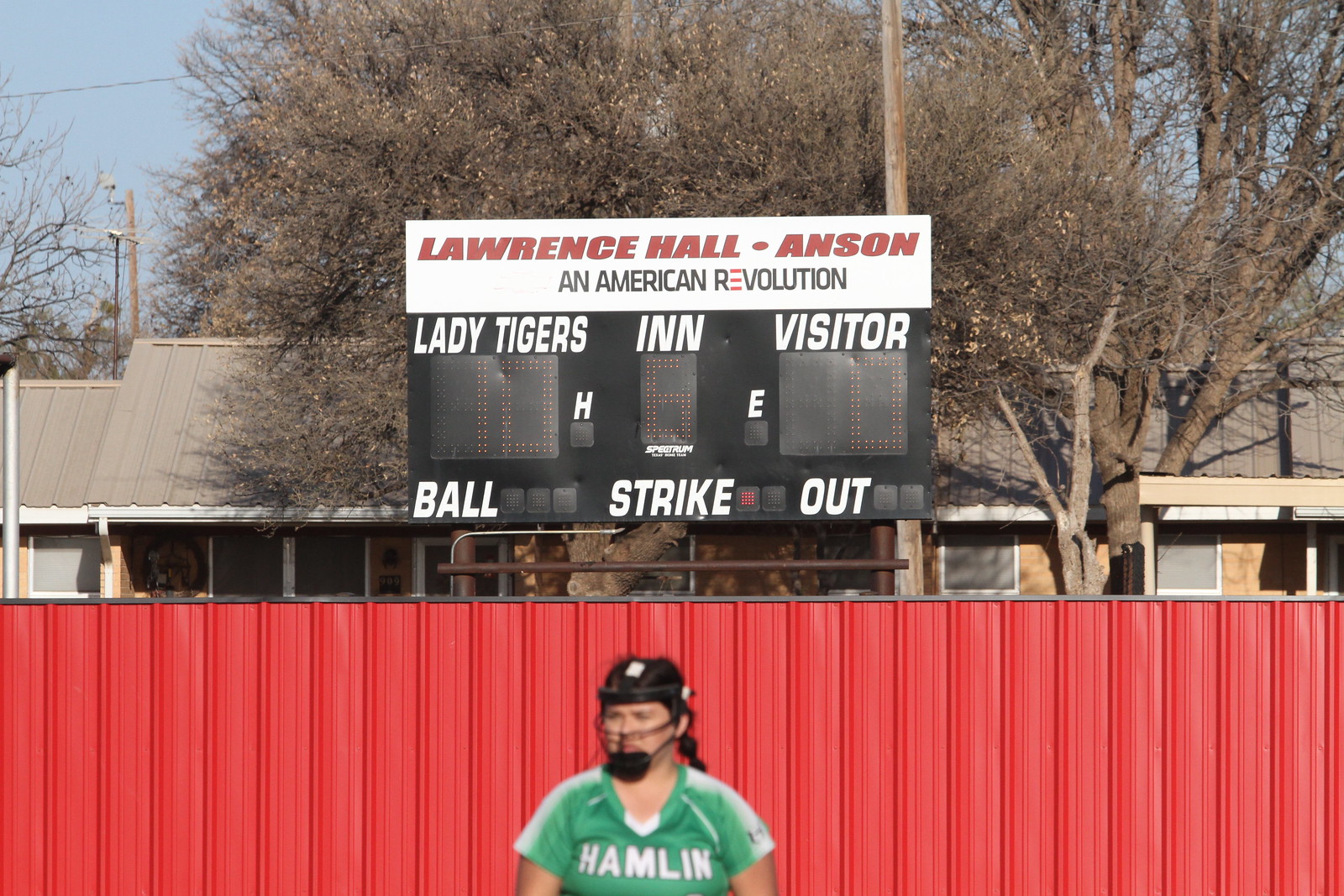In the image set against a blue daytime sky, a suburban neighborhood with brick houses and black rooftops forms the distant backdrop behind a vibrant green softball or baseball field. Dominating the scene is a prominent scoreboard that reads "Lawrence Hall-Anson" at the top, followed by "An American Revolution" in black lettering, with a distinctive red "E." Below, the digital section displays the Lady Tigers leading with a score of 10 against the Visitors' 0, currently in the 6th inning. Indicators show one strike, zero balls, and zero outs. At the bottom of the scene, a bright red fence lines the field, with a person wearing a green jersey with "Hamlin" in white letters and white sleeves visible in the foreground. The individual is also donning black headgear with a chin guard and face straps, ambiguously positioned—possibly a player or an umpire. To the left, a brown pole with white security cameras watches over the scene. Trees, showing signs of fall with bare branches, add a seasonal touch to this lively sports setting.